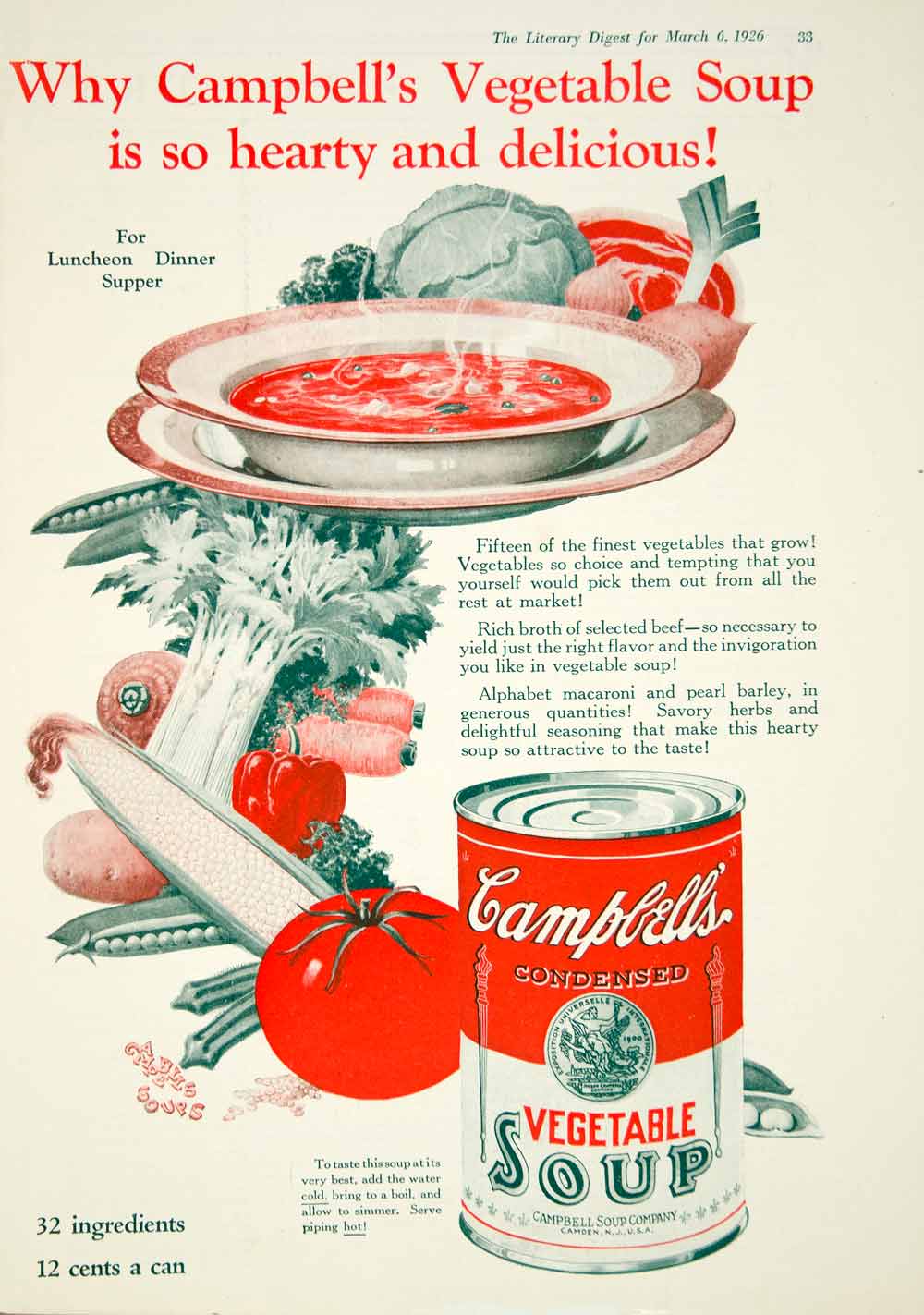The advertisement page showcases Campbell's Condensed Vegetable Soup with an intricate and vivid layout. Predominantly featuring a red and white Campbell's soup can with green text and a circular green logo, the can is positioned at the bottom right corner of the image. Central to the top portion of the page is a steaming bowl of bubbling hot red soup set in a ceramic bowl on a ceramic plate, flanked by an assortment of fresh vegetables including vibrant green broccoli, green peas, red tomatoes, orange carrots, and leafy cabbage. These vegetables are scattered towards the top center and left side, adding a colorful and fresh appeal. The background is a subtle grayish white, enhancing the vivid colors of the vegetables and soup. 

Text overlays the image, with a prominent heading in red at the top stating, "Why Campbell's Vegetable Soup is so hearty and delicious." Further details include information placed on the top right referencing "The Literary Digest for March 6, 1926." Additional text can be found to the right and bottom of the image, contributing to the overall narrative of the warmth and nutritious value of Campbell's soup. The careful placement of each visual and textual element makes this ad both informative and visually appealing, drawing attention to the wholesome qualities of the soup.